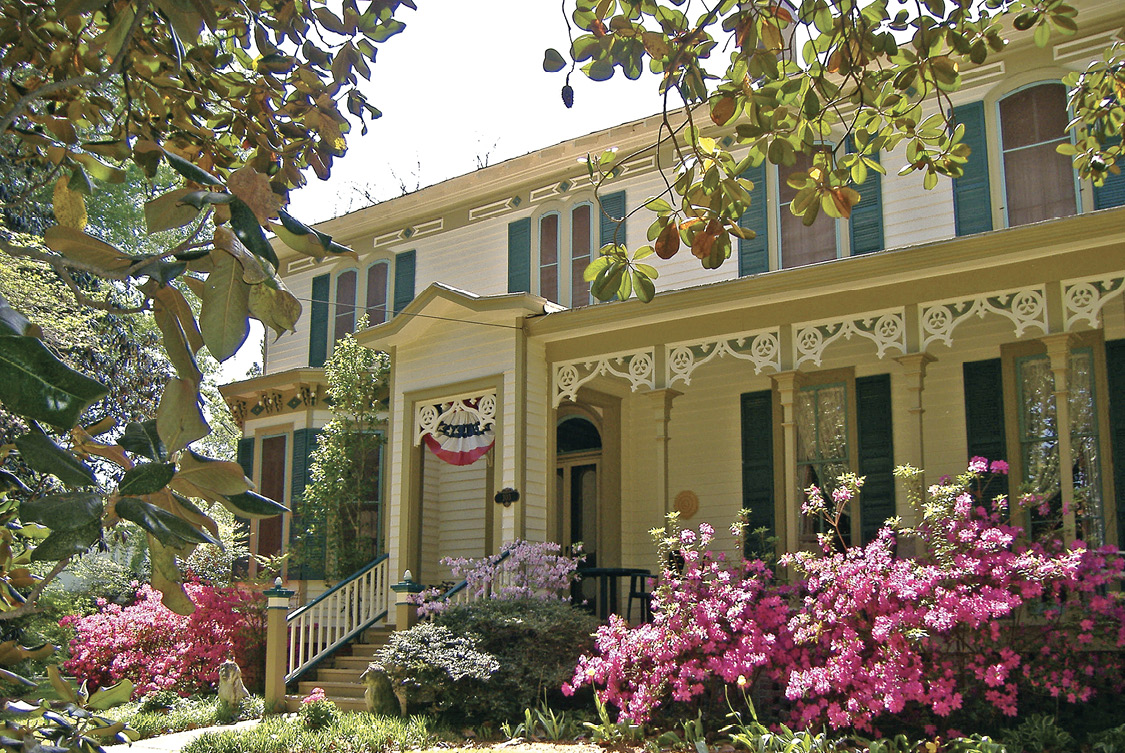This horizontally oriented photograph showcases a stately, two-story Victorian home that exudes classic charm and elegance. The house features a striking white facade complemented by mustard yellow borders and green shutters flanking the windows on both floors. The intricate woodwork around the porch, including delicate arches and lattice designs, adds to the home's vintage appeal. The expansive front porch, adorned with small wooden pillars and railings, invites visitors up a series of steps where a red, white, and blue sash hangs prominently at the main entrance. 

In the foreground, a well-tended garden bursts with the vibrant colors of late spring, displaying blooming shrubs and bushes with pink and purple flowers. The scene is framed by lush green grass and the overhanging branches of trees on both sides of the photograph, creating a serene canopy. The image captures a grounded perspective as if taken from beneath a tree, looking upwards into the clear sky, highlighting the grandeur and charm of this timeless residence.